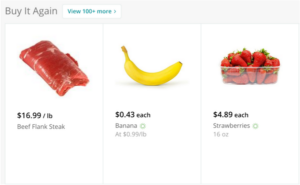The top of the image features a light gray banner. In the left corner, it displays the text "Buy it again." On the right side, in small blue text, it reads "View 100% more." Below this banner is a vibrant image of a raw red piece of meat labeled as "Beef Flank Steak" in light gray text with a price of $16.99 per pound ("$16.99 / LB"). To the right of the meat is a yellow banana priced at $0.43 each ("$0.43 each, Banana"). Further to the right, there is a small, clear plastic container filled with strawberries, each fruit displaying a green top. The strawberries are priced at $4.89 per container ("$4.89 each, Strawberries") with an additional note below indicating the weight as "16 OZ" (16 ounces).